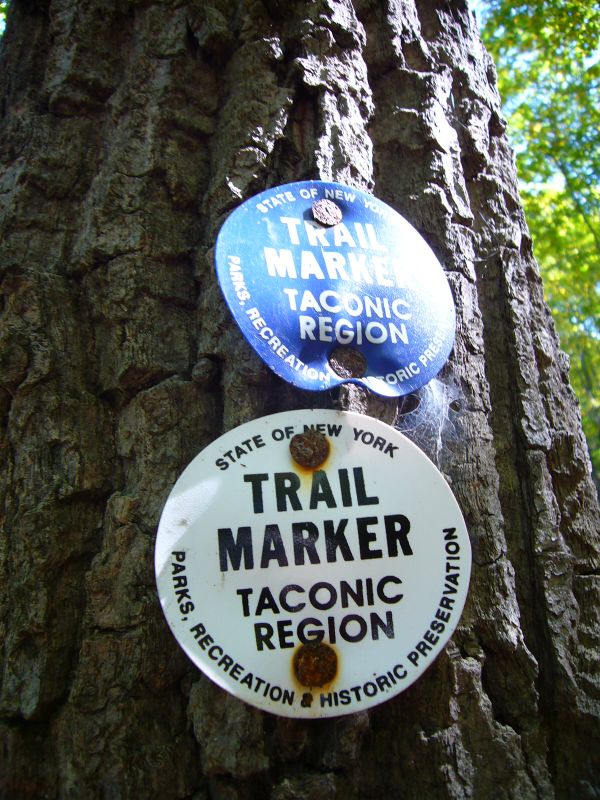This image captures a close-up view of two circular trail markers nailed to the gnarled bark of an old tree trunk, which dominates most of the photograph. The foliage in the background is minimal, with a slight wedge of high foliage visible to the right. Set in the Taconic Region of New York, these markers are designated for hiking trails. The top marker features a blue background with white text reading "Trail Marker Taconic Region" along with "Parks, Recreation, and Historic Preservation." The bottom marker is white with black text, displaying "State of New York" at the top, "Trail Marker Taconic Region" in the center, and "Parks, Recreation, and Historic Preservation" curving across the bottom. Subtle rust stains from the nails securing the markers are visible, adding character to the scene.